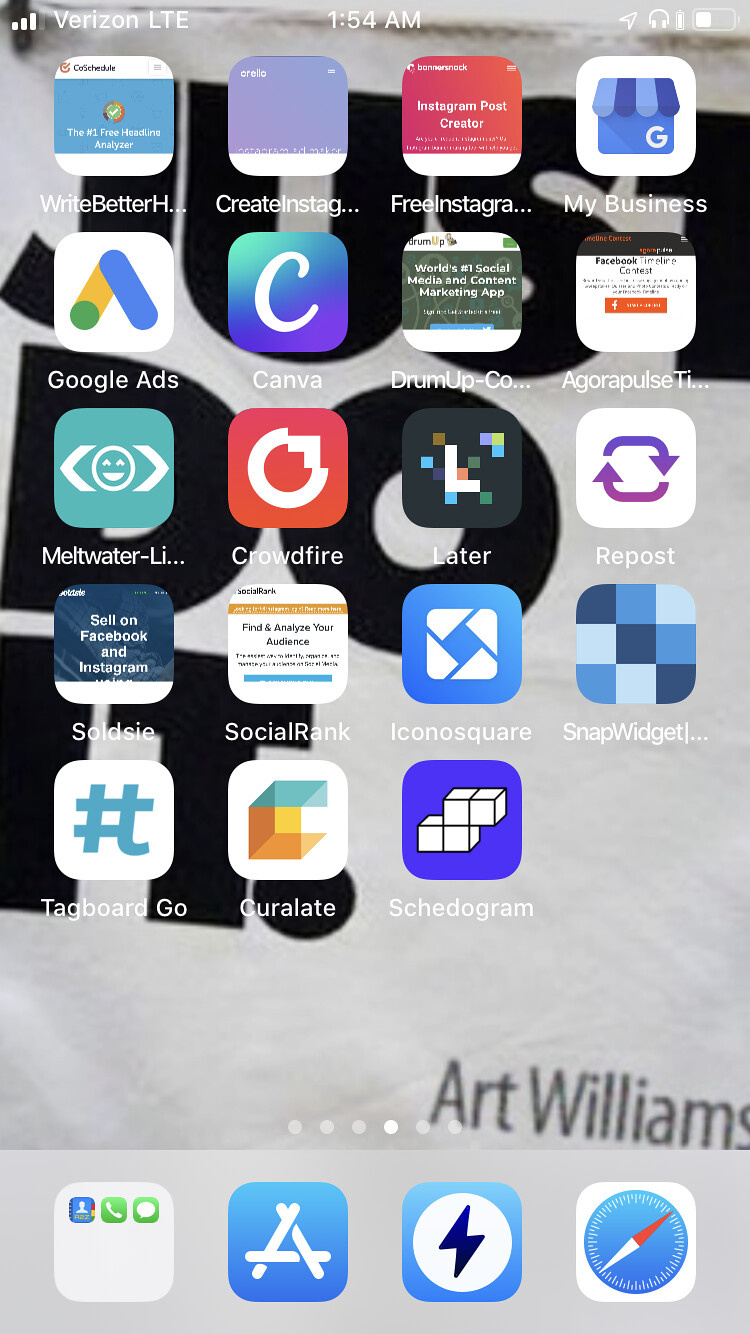The image captures the design of a smartphone home screen, prominently displaying various applications against a visually striking background. The background features the motivational text "just do it" in bold black letters, set on a light gray backdrop. In the bottom right corner, the name "Art Williams" appears in gray text.

At the bottom of the phone screen, there is a square containing three unspecified apps. To the right of this square is a blue icon with the letter "A," followed by a blue square featuring a blue lightning bolt. Next to this is the Safari logo, which consists of a white square with a blue circle and a compass in the center.

Above this row, the screen displays several app names in sequence: "Schedogram," "Guralate," "Tagboard Go," "SoldSea," "SocialRank," "Iconosquare," "SnapWidget," "Repost," "Loader," "Crowdfire," and "Meltwater." 

On the very top row, starting from the left, the apps are: "Google Ads," "Canva," "DrumUp," "Agorapulse," "MyBusiness," "FreeInstagram," "CreateInstagram," and "YsBetter." These elements together create a comprehensive and intricate layout for the smartphone home screen.